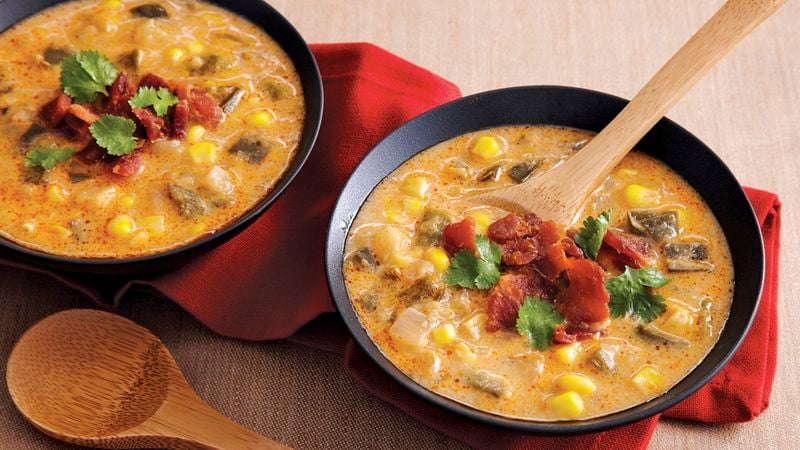This professional photograph captures two black bowls containing a vibrant, orange-hued soup or stew, likely an orange cream bisque or a curry coconut dish. The flavorful concoction features visible ingredients such as yellow corn kernels, possibly mushrooms, cilantro leaves, and an unidentifiable red component, possibly bacon. The bowl on the right is fully within the frame and has a wooden spoon resting inside it, while the partially visible bowl on the left lacks a spoon. Both bowls rest atop a fabric red napkin placed on a light brown table, which might be wooden. Additionally, another wooden spoon lies at the bottom left of the composition.